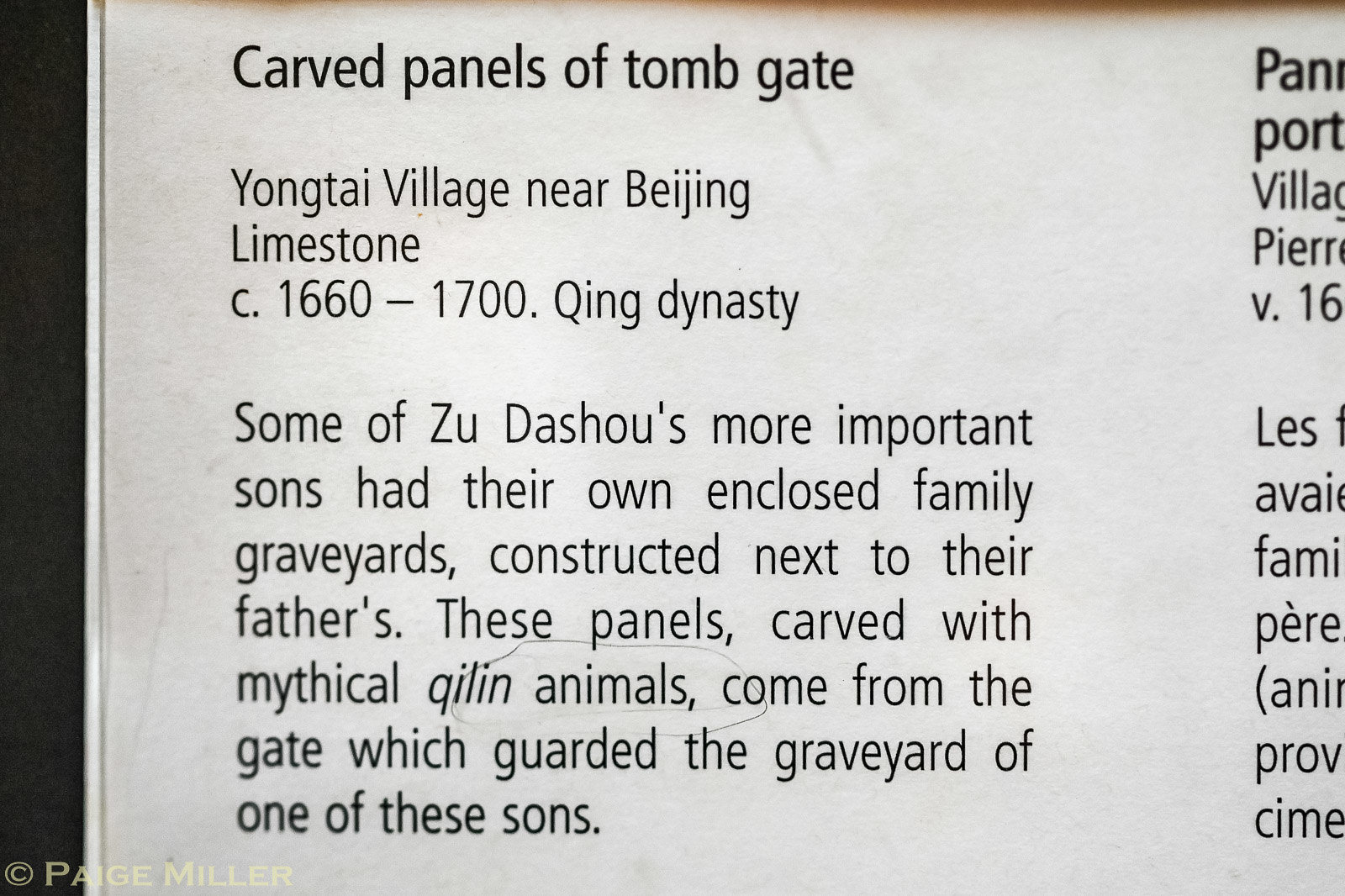The image shows a close-up photograph of an informational plaque or page, likely from a museum or exhibition manual. The title "Carved Panels of Tomb Gate" is prominently displayed at the top in a large, thin black font. Beneath the title, in a standard black font, it reads: "Yongtai Village near Beijing, Limestone, 1660 to 1700, Qing Dynasty." The text provides historical context, explaining that some of Zhu Daxiao's significant sons had their own enclosed family graveyards constructed next to their father's. These panels, intricately carved with mythical Qilin animals, were part of the gate guarding one such graveyard. The bottom of the image features a watermark in yellow letters reading "© Paige Miller." On the right-hand side, there is a glimpse of a similar paragraph in French, indicating the bilingual nature of the informational material.